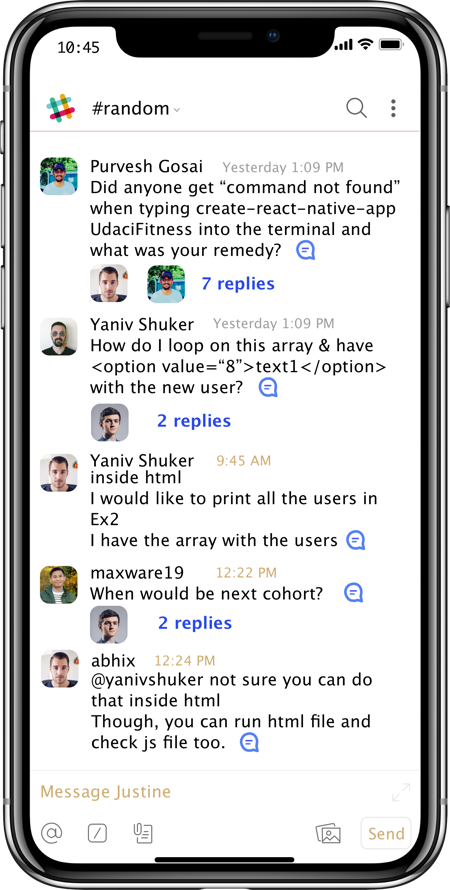The image showcases a mobile phone displaying a detailed chat interface. The phone's status bar indicates that the time is 10:45, with four bars of signal strength, a Wi-Fi connection, and a full battery. At the top of the screen, there is a hashtag icon laying on its side in blue, yellow, and red colors, labeled "#random" alongside a dropdown arrow. Near it are a magnifying glass icon and a vertical ellipsis (three dots stacked vertically).

The main focus of the screen is a chat conversation in a messaging app. The first message is from an avatar that appears to represent an Indian man named Purvish Gosai, posted at 1:09 p.m. the previous day. He asks, "Did anyone get 'command not found' when typing 'create react native app UDACI fitness' into the terminal, and what was your remedy?" Below his message is a speech bubble and two icons indicating there are replies.

Next, Yaniv Shukur, with another avatar image, responds at 1:09 p.m. the same day, "How do I loop on this array and have `<option value="8">Text One</option>` with the new user?" This message also has a speech bubble associated with it.

Yaniv Shukur continues the conversation at 9:45 a.m., stating, "Inside HTML, I would like to print all the users in 'ex2'; I have the array with the users." This message also displays a speech bubble indicative of replies. 

Then, Maxware joins the discussion at 12:22 p.m. asking, "When would be the next cohort?" His message includes two replies and a speech bubble.

Following up, another user named Abhix addresses Yaniv Shukur, saying, "@Yaniv Shukur, not sure you can do that inside HTML, though you can run the HTML file and check the JS file too." This brings us to additional interface elements such as a prompt to "Message Justine" in light peach-colored text, an @ symbol in the bottom corner, a box with a forward-slash, a paper icon with a paper clip, a photo icon, and an adjacent send button.